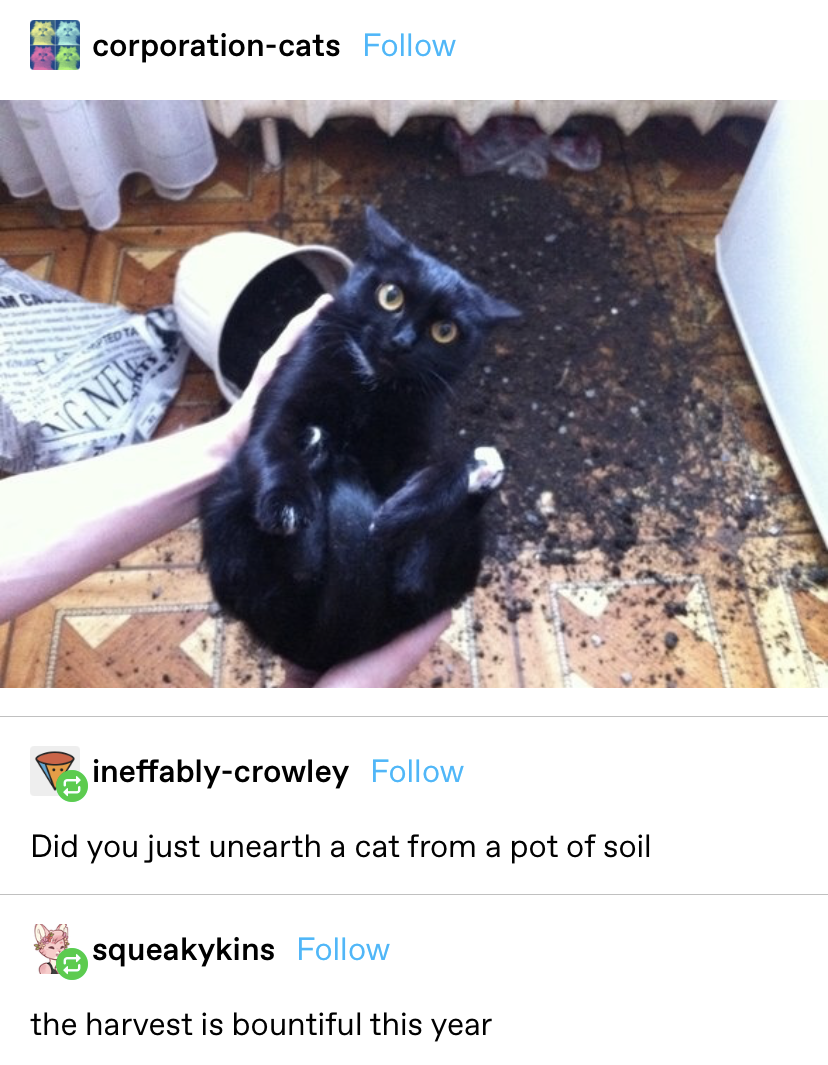The image is a detailed screenshot from a social media platform, prominently featuring a user named 'corporation.cats' whose profile icon showcases four colorful cat heads in yellow, blue, green, and pink. Adjacent to the profile name is a blue 'follow' button. The main focus of the photograph is a black cat with yellow eyes, being held belly up by two hands in the lower left corner. The cat stares directly at the camera with its ears pointed downwards, looking distinctly unhappy. Scattered around the wooden floor are spilled dirt and a tipped-over plant pot, suggesting the cat's mischievous act. The background includes a white radiator, curtains, and a bag with a newspaper-like design. Below the image, comments from users 'ineffably-crowley' and 'squeakykins' add to the humor with the remarks, "Did you just unearth the cat from a pot of soil?" and "The harvest is bountiful this year." The setting emphasizes the chaotic aftermath and the cat's innocent but guilty expression.